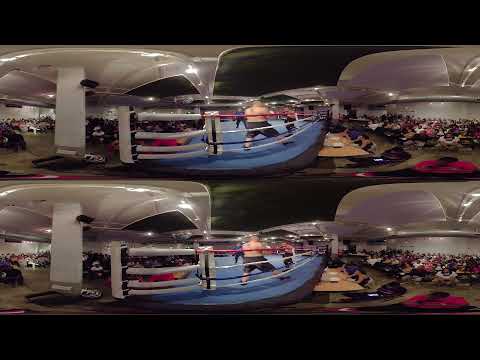The image showcases a duplicated panoramic photograph, each replication placed one on top of the other, bordered by thick black lines at both the top and bottom. The central focus of the panoramic image is a boxing stage set on a blue ground with a red, white, and black fence pattern, consisting of four ropes—red at the top, followed by white, dark blue, and white at the bottom. Dominating the foreground is a boxer in black shorts with his back visible, facing an opponent dressed in a red top and black pants. A referee dressed in white is visible walking at the far end of the stage, while a large audience occupies the right part of the image.

The image appears to be arranged into two rows with three columns, presenting the same distorted and stretched-out photographs in each section, making the details within them somewhat challenging to discern. The leftmost segment hints at a parking lot with visible cars and a white pillar stretching from the floor to the ceiling. The middle segment amplifies the boxing scene, emphasizing the two boxers and the onlookers seated ringside near a wooden scores table. The right segment depicts an auditorium bustling with seated individuals. Overall, the detailed panorama captures a dynamic and immersive scene of a boxing match and its surrounding environment.